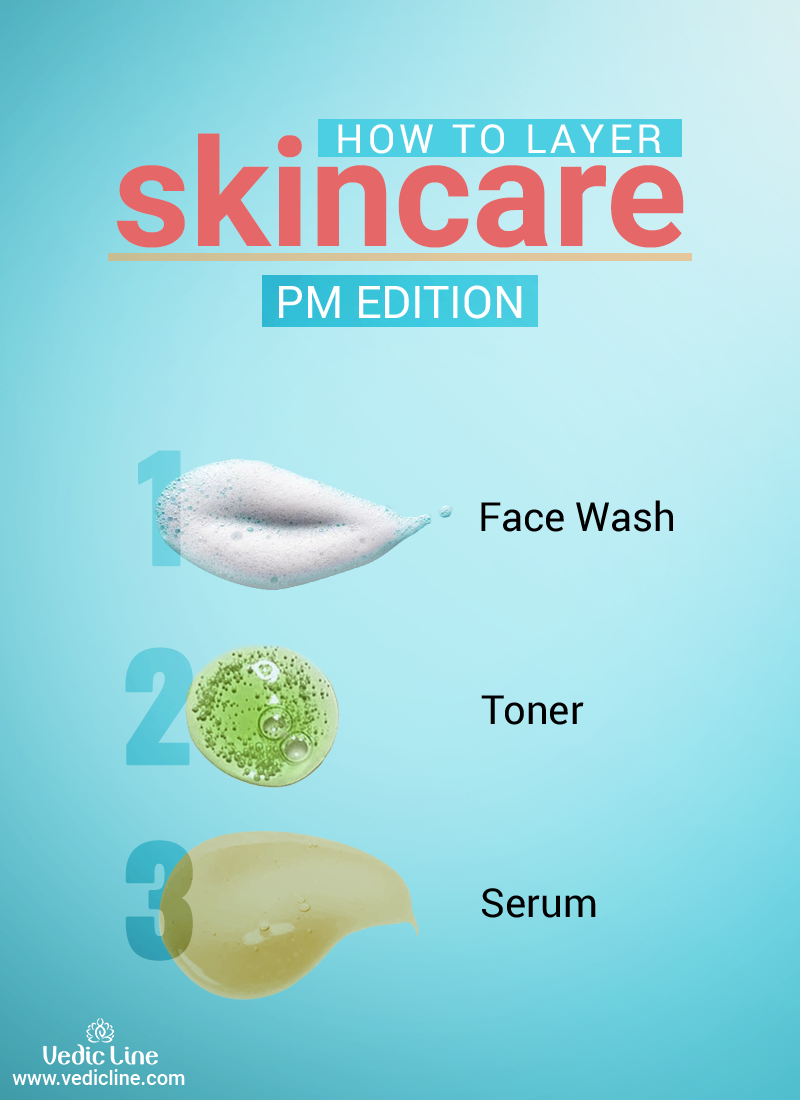The advertisement for VedicLine is set against a gradient background that transitions from a whiter shade in the upper right corner to a light blue towards the bottom. Dominating the top portion, white letters announce "How to Layer" with "Skincare" highlighted in bold red letters underneath. Below this, an orange-yellow bar underscores the text, which is followed by the subtitle "PM Edition." 

The centerpiece of the advertisement features three products arranged vertically, each accompanied by both a visual representation and label. The first product is a white foamy face wash, marked as "1. Face Wash" with a shadowed numeral beside it. The second product is a green toner with microbeads labeled "2. Toner." The third product is a tawny brown serum, slightly translucent, denoted as "3. Serum."

In the bottom left corner, the name "VedicLine" is displayed, followed by their website "www.vedicline.com." The advertisement's layout effectively guides the viewer through the recommended skincare layering process using VedicLine products.